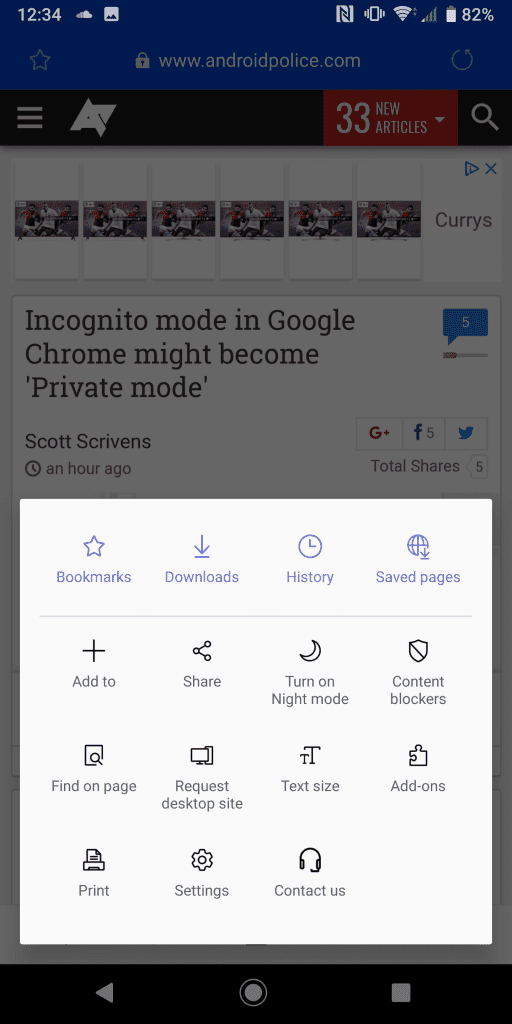The image displays a vertical cell phone screen showing a webpage from www.androidpolice.com at the top. Just below the URL, there's a notification indicating "33 new articles." One of the articles is highlighted with the headline: "Incognito mode in Google Chrome might become private mode."

Superimposed on this webpage is a semi-transparent white overlay that occupies the upper portion of the screen. At the top of this overlay, there are the tabs: "Bookmarks," "Downloads," "History," and "Saved Pages." Below these tabs, a horizontal line separates this section from the rest of the overlay, which contains multiple options organized in a list. These options are: "Add to," "Share," "Turn on Night Mode," "Content Blockers," "Find on Page," "Request Desktop Site," "Text Size," "Add-ons," "Print," "Settings," and "Contact Us." Each option is enclosed in a distinct white box.

The underlying cell phone screen beneath this white overlay has been grayed out, indicating that the overlay is currently active. 

At the top of the screen, the device status bar is visible, showing a time of 12:34, a battery level at 18%, and an active WiFi connection.